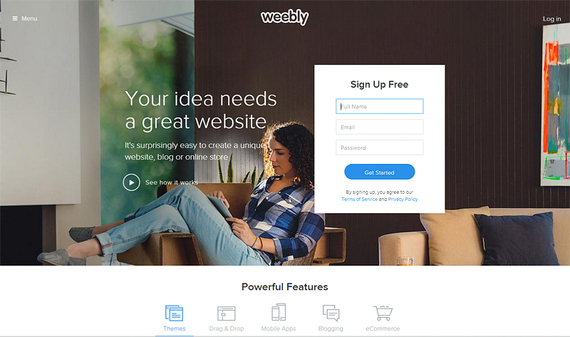The top section of a website prominently features a visually engaging image. On the right-hand side, part of a beige sofa with two pillows—one beige and one black—is visible. Adjacent to the sofa is a brown wall adorned with an abstract painting, featuring streaks of green, grey, red, and yellow. Above the painting, the word "Login" is written in white.

The scene transitions to a white wall on the other side of the frame, where a woman is seated. She is dressed in blue jeans and a blue and white checkered shirt, accessorized with suspenders. She appears to be focusing on something in her lap, possibly a handheld device or document, giving the impression of being occupied.

Above the woman, the caption in white reads, "Your Idea." A subheadline follows: "It's a great website. It's surprisingly easy to create a unique website, blog, or online store." Below this, there is an outlined white circle with a white rectangle inside, accompanied by the text, "See How It Works."

At the very top of the page, the brand name "Weebly" is displayed in white against a darker background. Below this, a prominent white rectangle contains the call-to-action "Sign Up For Free" in black lettering. The registration form includes input boxes with blue and grey outlines, labeled "Full Name," "Email," and "Password." The section concludes with a blue oval button containing the white text, "Get Started."